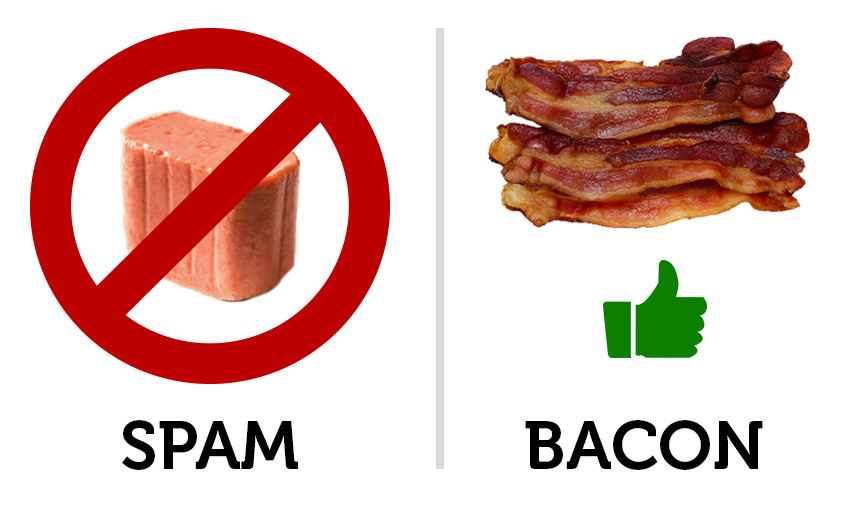In this landscape-oriented image, set against a white background, a clear comparison between two food items is illustrated. The image is divided into two columns by a thin vertical gray line. On the left side, there's a piece of Spam, still in its canned shape, overlaid with a thick red circle and diagonal red line, indicating disapproval. Below the Spam, black text reads "Spam." On the right side of the gray line, three freshly cooked strips of bacon, displaying a rich blend of red meat and white fat, are stacked horizontally. Beneath the bacon, a green thumbs up symbol suggests approval, complemented by black text that reads "Bacon." The dominant colors include shades of red, pink, white, black, and green. The overall message, enhanced by the visual symbols and text, clearly conveys a preference for bacon over Spam.